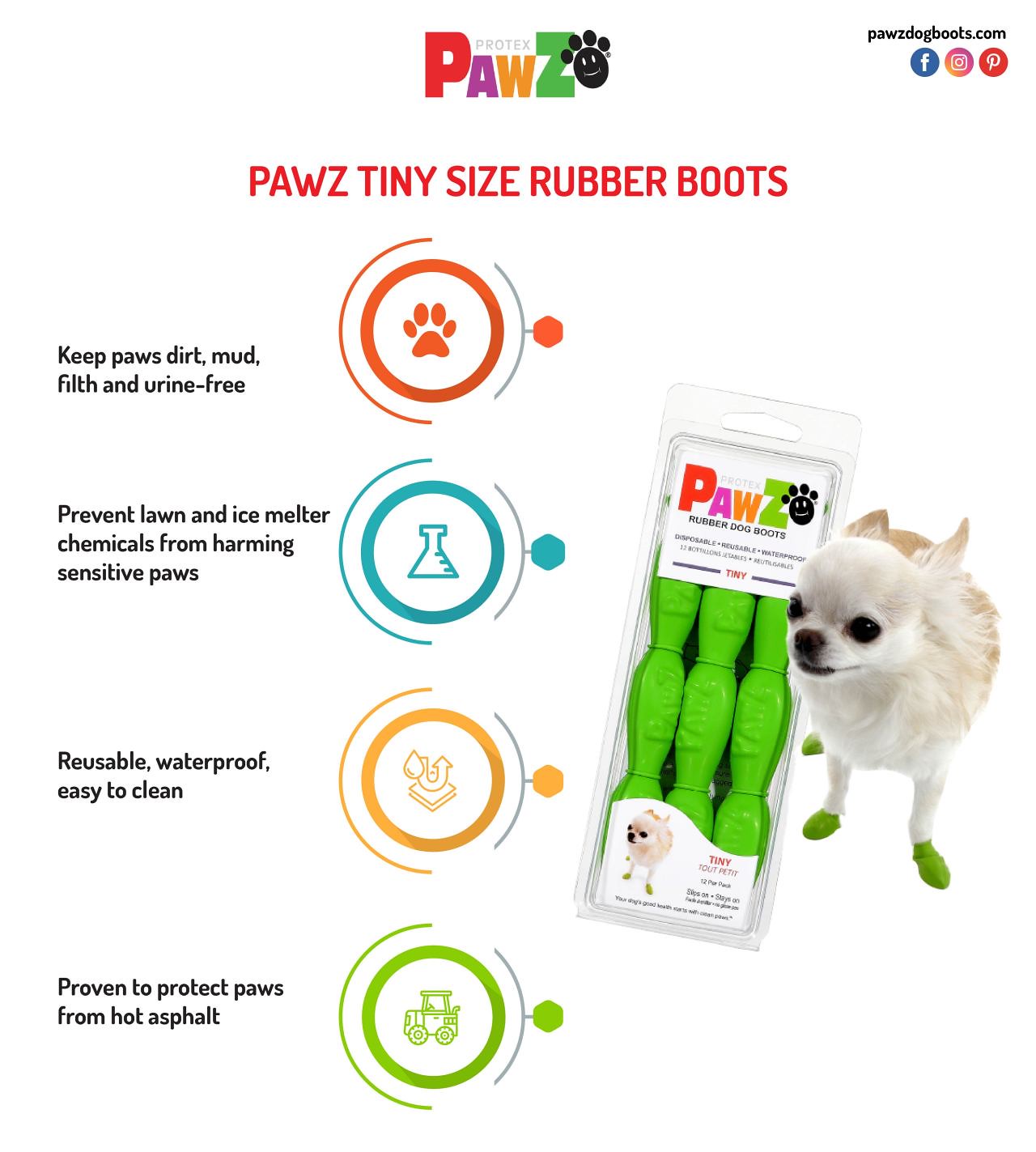The advertisement for Protex PAWZ Tiny Size Rubber Boots features a colorful and engaging design aimed at showcasing the benefits and appeal of the product. The brand name "P-A-W-Z" is prominently displayed in large, multicolored letters, with 'P' in red, 'A' in purple, 'W' in orange, and 'Z' in green. Beneath this vibrant logo, the text "Paws Tiny Size Rubber Boots" is written in red font.

A key visual component of the ad is a charming image of a small Chihuahua, adorned with green rubber boots on its paws, adding a cute and practical touch to the presentation. The packaging of the product also features prominently, showing three of the tiny green rubber boots through a clear plastic casing.

On the left side of the advertisement, there are four distinct icons that elaborate on the product's benefits:

1. A red icon of a paw print, accompanied by the text: "Keep paws dirt, mud, filth, and urine free."
2. A blue icon of a laboratory beaker, with the text: "Prevent lawn and ice melter chemicals from harming sensitive paws."
3. An orange icon resembling cleaning wipes, detailed with the text: "Reusable, waterproof, easy to clean."
4. A green tractor icon with the text: "Protect paws from hot asphalt."

These highlights emphasize the practicality and protective features of the PAWZ rubber boots. Additionally, the top right corner of the advertisement includes a URL (pawsdogboots.com) and social media icons, providing further avenues for interaction and purchase. This detailed yet vibrant advertisement effectively communicates the utility and charm of PAWZ Tiny Size Rubber Boots for your beloved pet.